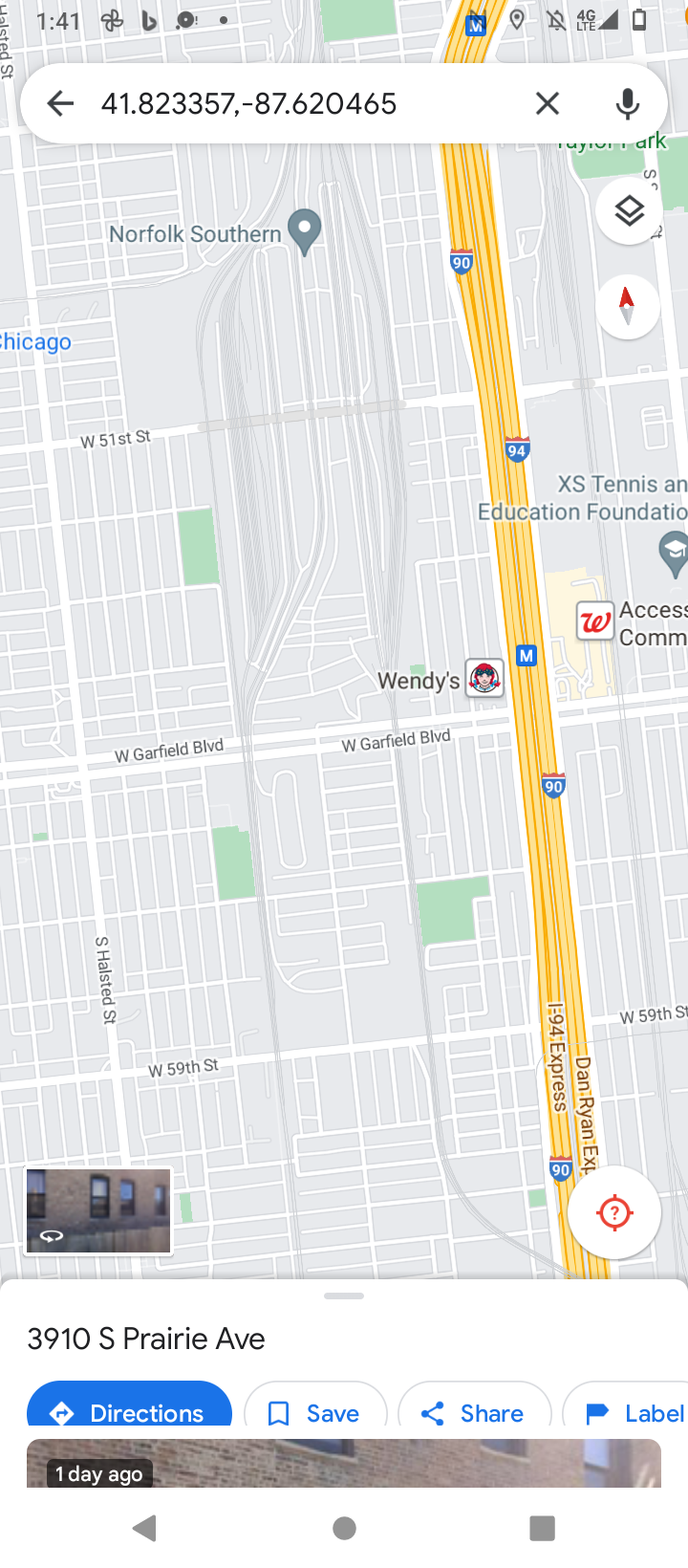The image displays a detailed navigation map from a smartphone, pinpointing the exact coordinates 41.823357, -87.620465. In the top left corner, several icons are visible: a ‘1,41’ designation, a pinwheel shape, an unrecognized symbol, and a circle encircled by two small dots. On the far right, a few more icons appear, including an unrecognizable symbol, a navigation pin, a bell with a slash through it indicating notifications are silenced, a '4G LTE' network signal indicator, a full bar signal strength icon, and a mostly depleted battery symbol.

At the bottom of the map, the coordinates lead to 3910 South Prairie Avenue. There is a blue button labeled 'Directions' in white text, and to its right, a white button with blue text that says 'Save'. Another button labeled 'Share', represented by three dots connected by lines, follows. Near these buttons is a white circle bearing a blue text label, and adjacent to it is a flag with a small label.

Prominently in the middle bottom-left portion of the image is a street-level view of the location. The map details surrounding areas with notable features such as the 90 Freeway, 'Blue Shield', and 'Red Top'. The map also marks various streets, including 'West Scarfield Boulevard', where a Wendy’s restaurant is located near the freeway. Other visible streets are '59th Street', 'South Something Street', and a label in blue text that says 'Chicago'.